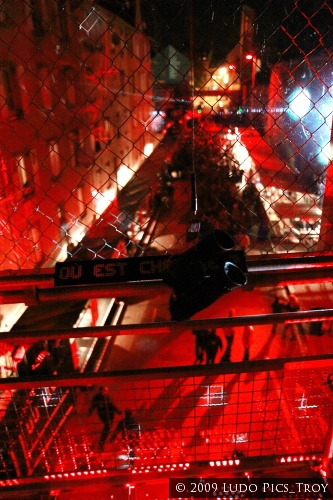This photograph captures a vibrant, nighttime cityscape from an elevated vantage point, likely from a pedestrian bridge or balcony. The viewer's perspective is from behind a metallic fence that spans the center of the image, acting as a visual barrier between the camera and the bustling street below. The street is bathed in a striking red hue, emanating from numerous lights that illuminate the area. Below, people are visible walking along the sidewalks, and various street vendors add to the dynamic atmosphere. The road is flanked by tall buildings, each adorned with countless windows that reflect the crimson glow of the streetlights. The sky overhead is a deep black, contrasting sharply with the vivid street scene. In the bottom right corner, a white text watermark reads, "© 2009 LudoPix_Troy." Additionally, partially obstructed white text on a railing spells out "D-U-E-S-T-C-H-A," hinting at the possible name of the location captured in this striking image.